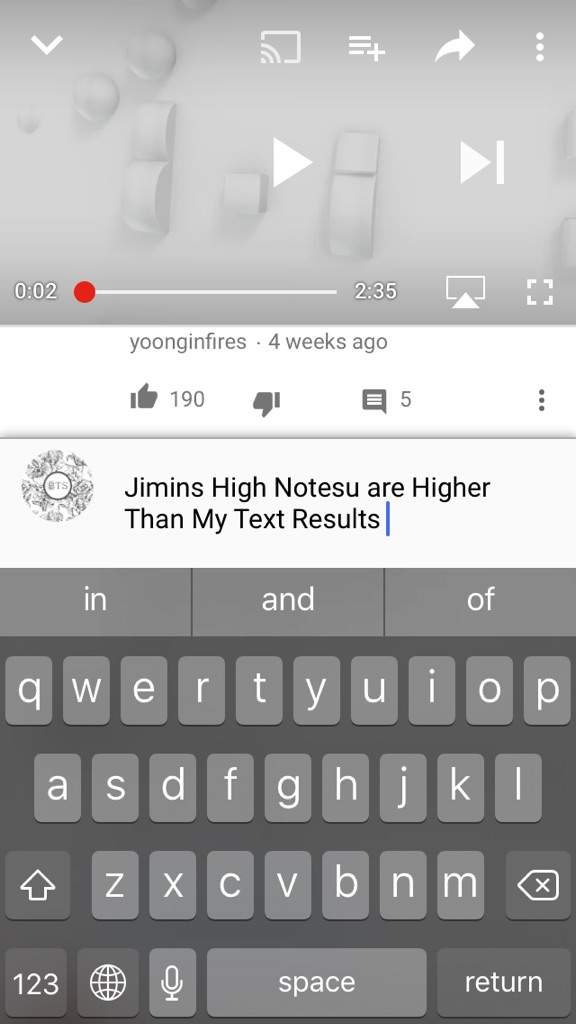Screenshot of a tablet displaying a text input interface, with the virtual keyboard occupying the bottom half of the screen. The keyboard layout includes the standard QWERTY arrangement: "QWERTYUIOP" on the first row, "ASDFGHJKL" on the second row, and "ZXCVBNM" on the third row. Next to "Z" is a shift key, while a backspace key is positioned to the right of "M". Additional keys along the bottom include a "123" key for numeric input, a globe icon for language settings beneath "Z", a microphone icon beneath "X", a space bar beneath "C", "V", "B", and "N", and a return key beneath "M" and the backspace key.

At the top of the screen, there are predictive text options suggesting the words "in", "and", and "of". In the middle of the screen, the text reads: "Jimens, hi, notesu, are higher than my text results." This is explicitly spelled out as "Jimens" (J-I-M-I-N-S), "hi" (H-I-G-H), and "notesu" (N-O-T-E-S-U).

Above the text, a comment is visible, posted by "YoongiMfires" (Y-O-O-N-G-I-M-F-I-R-E-S) four weeks ago, followed by a thumbs-up icon with 190 engagements, a thumbs-down icon with no engagements, five comments, and a menu represented by three dots for more options.

At the very top, there is an interface element resembling a play button, indicative of a video, currently paused at 2 seconds with a total duration of 2 minutes and 35 seconds.